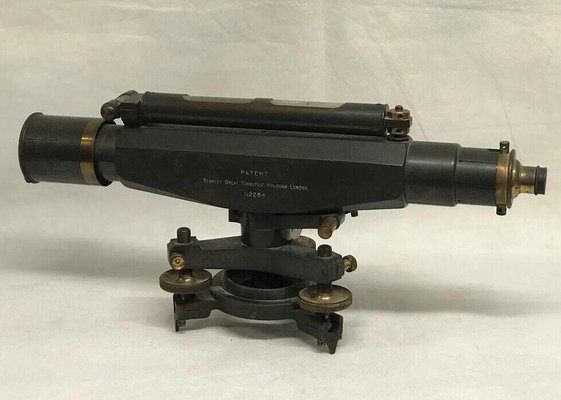The image depicts an antiquated, rusted optical scope, likely designed for attachment to a firearm or similar instrument. The scope features a pronounced eyepiece on the right-hand side, intended for an individual to set their eye against. On the opposite end, the left-hand side, the scope widens slightly to accommodate a lens. The entire device exudes an aged aesthetic, its surface cloaked in a near-black patina that suggests it could be rusted iron or bronze. The wear and oxidation on the scope hint at a long history, evoking a sense of vintage craftsmanship and durable design.